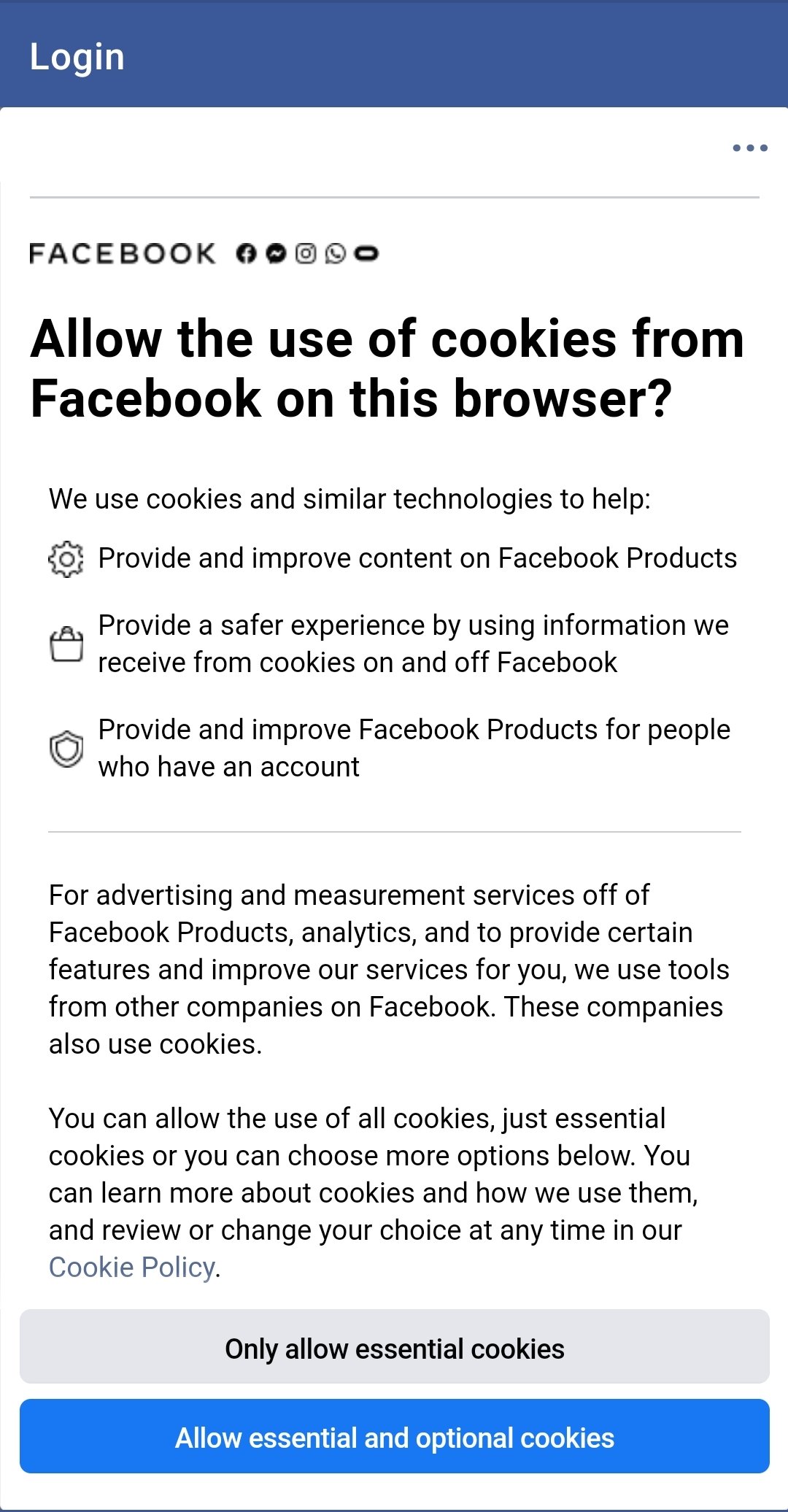The image depicts a Facebook login page displayed on a desktop browser. The screen prominently features a cookie consent prompt from Facebook. There are two noticeable buttons: a gray button labeled "Allow essential cookies only" and a blue button labeled "Allow essential and optional cookies." The prompt informs users about the purposes of these cookies, including the provision and improvement of content and Facebook products. Essentially, it highlights how Facebook seeks consent to use cookies, which enables the platform to collect user data and tailor content and advertisements based on user preferences. This practice aligns with Facebook's well-known approach to handling user information and targeted advertising.